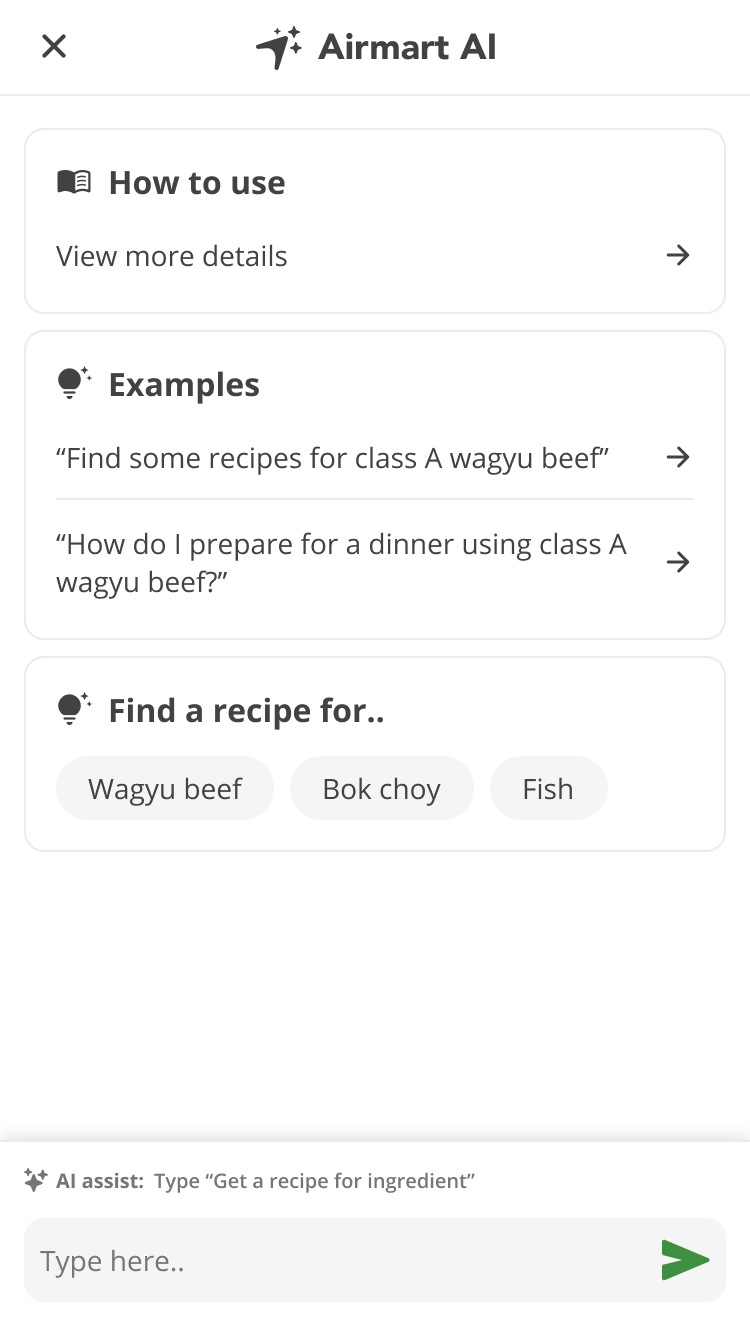The image depicts a screenshot of a white vertical rectangular box with various elements arranged systematically. 

At the top left corner, there is a black 'X' icon. Centrally positioned at the top is an arrow or triangle pointing upwards, flanked by three stars. Below this icon, the text reads "Airmart" followed by "A-I-R-M-A-R-T" and "A-I". 

Below this header, there is a rectangular box with a gray highlighted border that contains the text "How to Use" accompanied by a booklet icon to its left. Directly underneath, there is the text "View more details" with a black arrow pointing to the right.

The next section is another rectangular box titled "Examples" featuring a light bulb icon on its left. The first example line reads, "Find some recipes for Class A wagyu beef," with a black arrow pointing to the right. The second example line states, "How do I prepare for a dinner using Class A wagyu beef?" followed by another right-facing arrow.

Following this, there is another rectangular box highlighted in gray with the heading "Find a Recipe for," accompanied by a light bulb icon to its left. This section includes three categories labeled under oval buttons: "Wagyu Beef," "Bok Choy," and "Fish."

At the very bottom of the box, there is an icon resembling a plus sign surrounded by two or three stars, with the text "AI Assist. Type 'Get a recipe for ingredient'." Adjacent to this, there is a search bar marked with the prompt "Type here" and a green arrow pointing to the right.